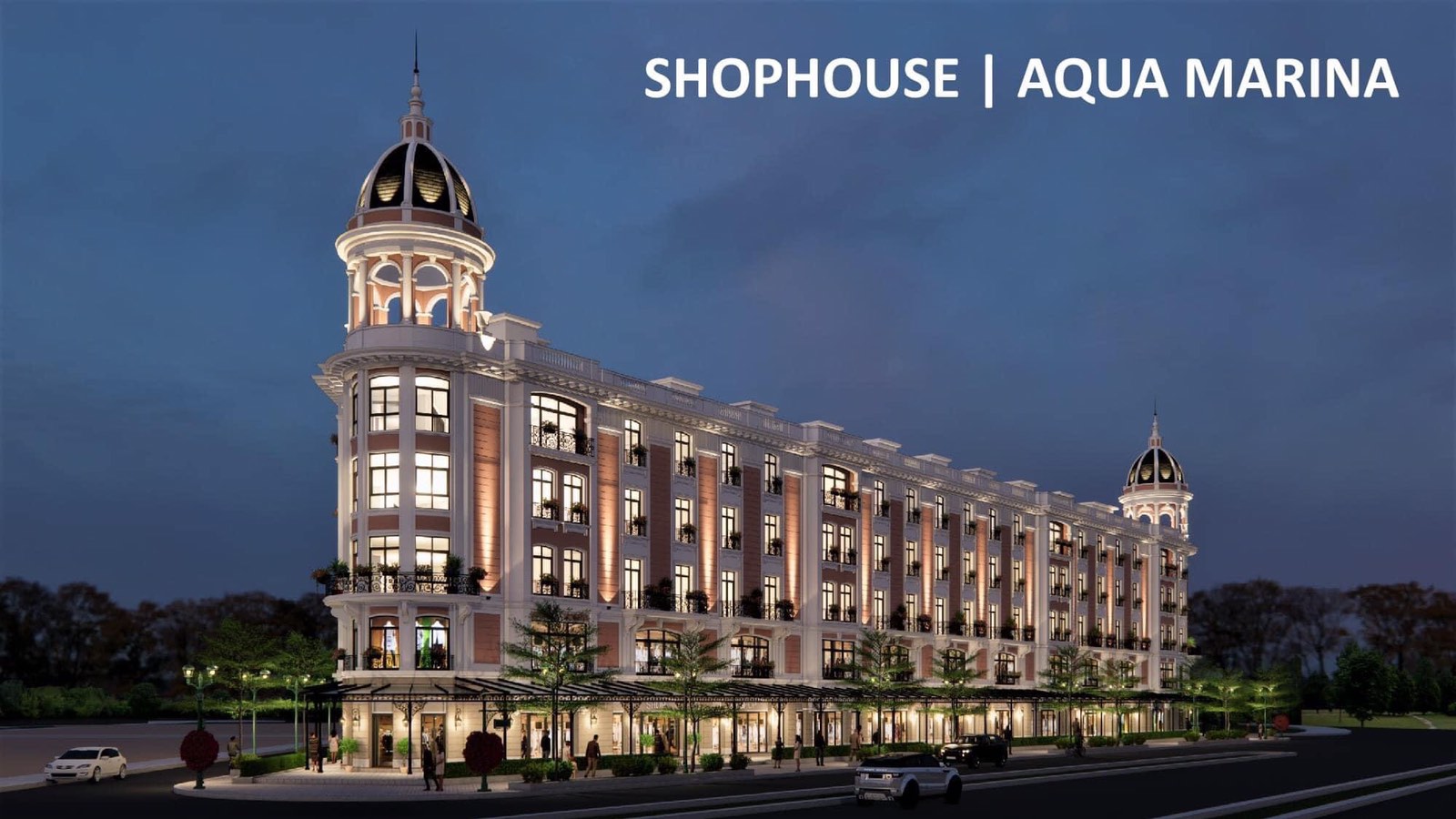The image showcases a bustling urban scene during the evening, featuring a prominently positioned multi-story building at the center. The building spans horizontally across the frame, with an estimated five to six floors, displaying numerous windows and small balconies adorned with plants. Notably, the roof includes two distinctive tower cupolas. 

At ground level, the structure likely houses shops, while the upper floors appear residential. Surrounding the building are trees, enhancing the lively atmosphere. On the streets below, two cars are visible, along with pedestrians walking on the sidewalks. The sky above transitions to a medium-dark blue with grayish clouds, adding to the twilight ambiance. 

In the top right corner of the image, bold white text reads, "Shop House Aqua Marina". The photograph is well-lit and has a vivid color palette including white, blue, brown, black, yellow, red, and green, giving it a vibrant, almost magazine-like quality.